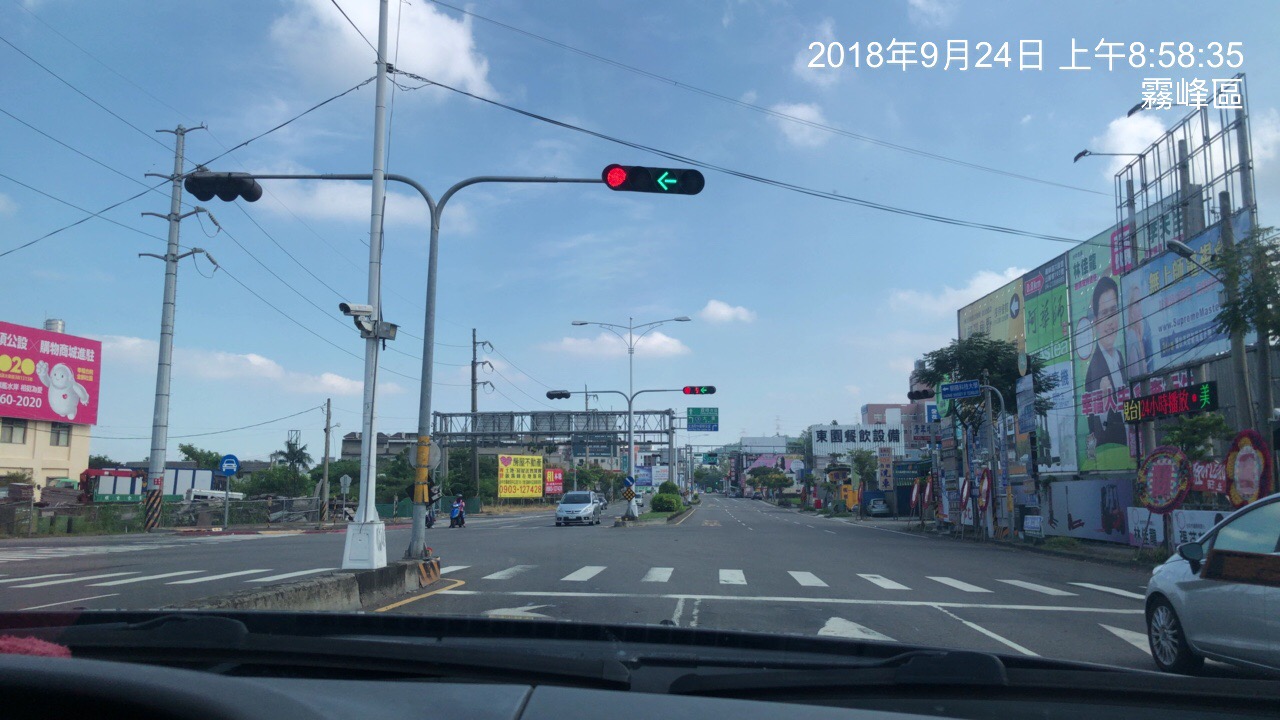The image captures a bustling city street scene in an Asian country, viewed from the perspective of a car with a dash cam approaching an intersection. The photograph was taken on a clear day, as evidenced by the blue sky with a few white fluffy clouds. The upper-right corner of the image displays a timestamp in white font, denoting the year 2018 followed by text in Chinese, Korean, or Mandarin, registering the time as 8:58:35.

The wide street features three lanes of traffic in each direction, with white road markings for crosswalks and turn arrows. A gray car is visible to the right, driving alongside the car with the dash cam. Another gray car is seen coming towards the intersection from the opposite side. Traffic lights are present, including a prominent red light and a green arrow indicating a left turn.

Lining the street are various signs and billboards adorned with vibrant colors and Asian script. On the left side, there's a notable pink billboard featuring a large white puffy character. More signage is visible on buildings to the right, including a black billboard with an Asian mascot and advertisements featuring an Asian man. These details collectively hint at a lively urban environment bustling with visual information and commercial activity.